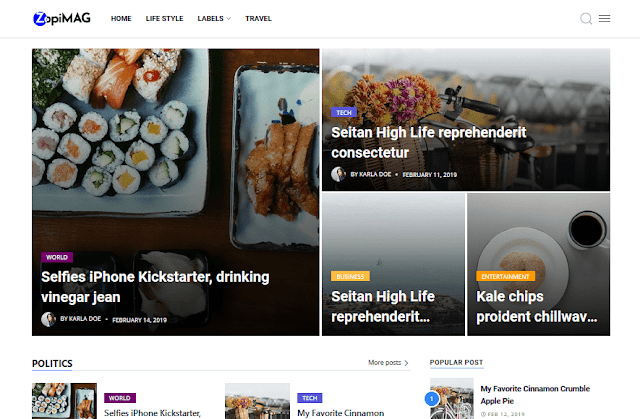The captured image is from a website displaying a variety of categories and articles. 

At the top of the page, the site’s title is prominently featured as "ZipMAG ZAPMAG," with "MAG" in uppercase letters. Adjacent to the title are navigational links for "Home," "Lifestyle," "Labels," and "Travel."

Below the navigation bar, there is a vibrant photograph of assorted sushi wraps arranged on a plate alongside some fish. Following this image, a series of article topics are listed: "World," "Selfies," "iPhone," "Kickstarter," "Drinking Vinegar," "Gene," and the date "February 14th, 2019."

In the "Tech" section, the articles include titles such as "Seaton," "High Life," "Reprehendent," "Turdent," and "Consecutor." For the "Business" category, the titles listed are "Seaton," "High Life," and "Repentateur."

Under "Entertainment," the articles mentioned are "Kale Chips," "Provident," "Chill," followed by ellipses.

Towards the bottom of the page, there are additional clickable links related to "Politics" and "Tech." Notable articles here include "My Favorite Cinnamon," "My Favorite Cinnamon Crumble Apple Pie," along with sections for "More Posts" and "Popular Posts."